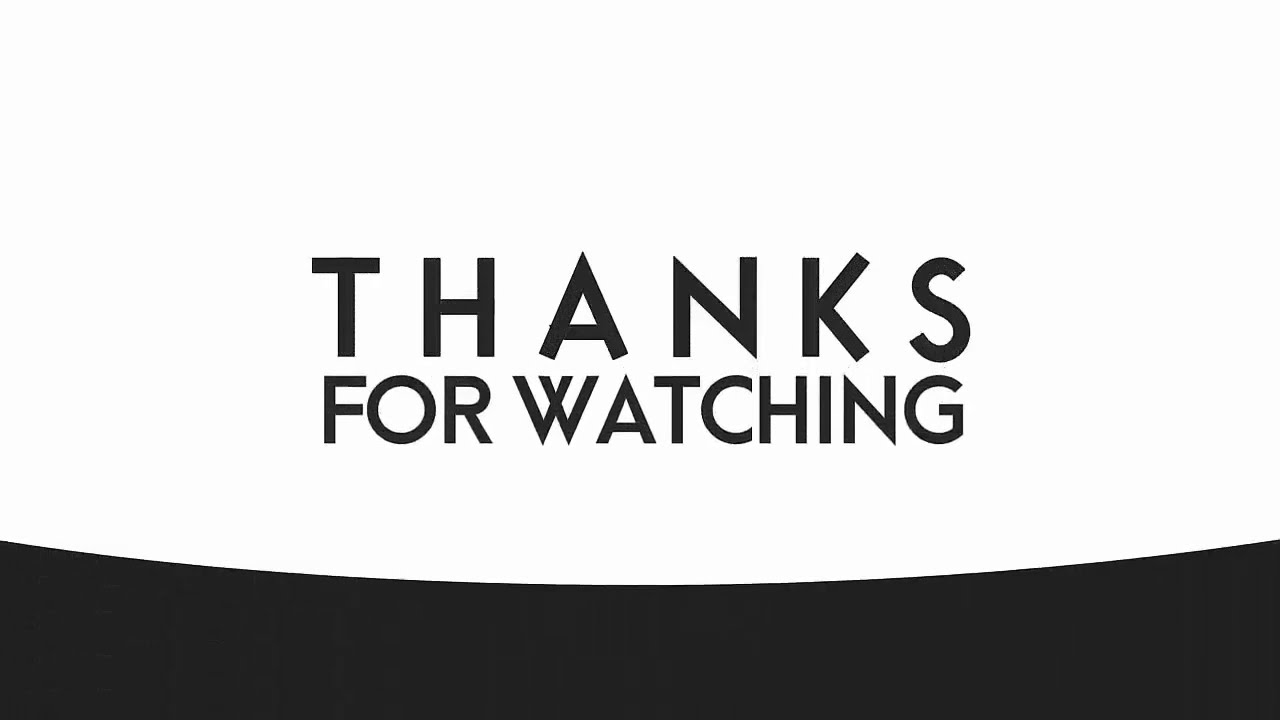The image features a text that reads "THANKS FOR WATCHING" in black capital letters, set against a white background. The word "THANKS" is positioned on the upper line with slightly more spacing between the letters, while "FOR WATCHING" is directly below it on a separate line with little to no spacing between the letters. At the bottom of the image, there is a black horizontal strip whose upper boundary curves gently upwards from one corner to the other, with the left and right ends slightly higher and the middle portion dipping lower. This design element gives the image a nostalgic feel, reminiscent of classic television shows from the 1950s to 1970s.